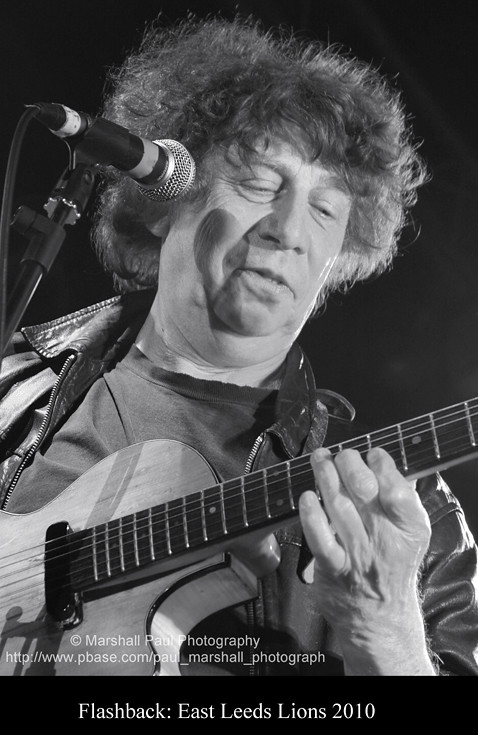In this captivating black-and-white portrait photograph, an elderly man with voluminous, fuzzy hair reminiscent of 80s rock band styles is passionately playing an electric guitar. The close-up shot, taken from a low angle, allows his head to dominate the upper part of the frame while his guitar-playing hand and part of the instrument fill the lower section. He seems to be enjoying the moment, potentially mid-song, with a black microphone featuring a mesh spherical tip pointed towards him, amplifying his voice. The man is dressed in a leather-ish jacket over a t-shirt, adding to his rockstar aesthetic. A watermark at the very bottom of the photograph credits "Marshall Paul Photography" and includes a URL link, "http://www.pbase.com," along with a © trademark icon. Below this watermark, a black border contains the inscription "Flashback: East Leeds Lions 2010" in white text, possibly referencing the name of the band from East Leeds, England.